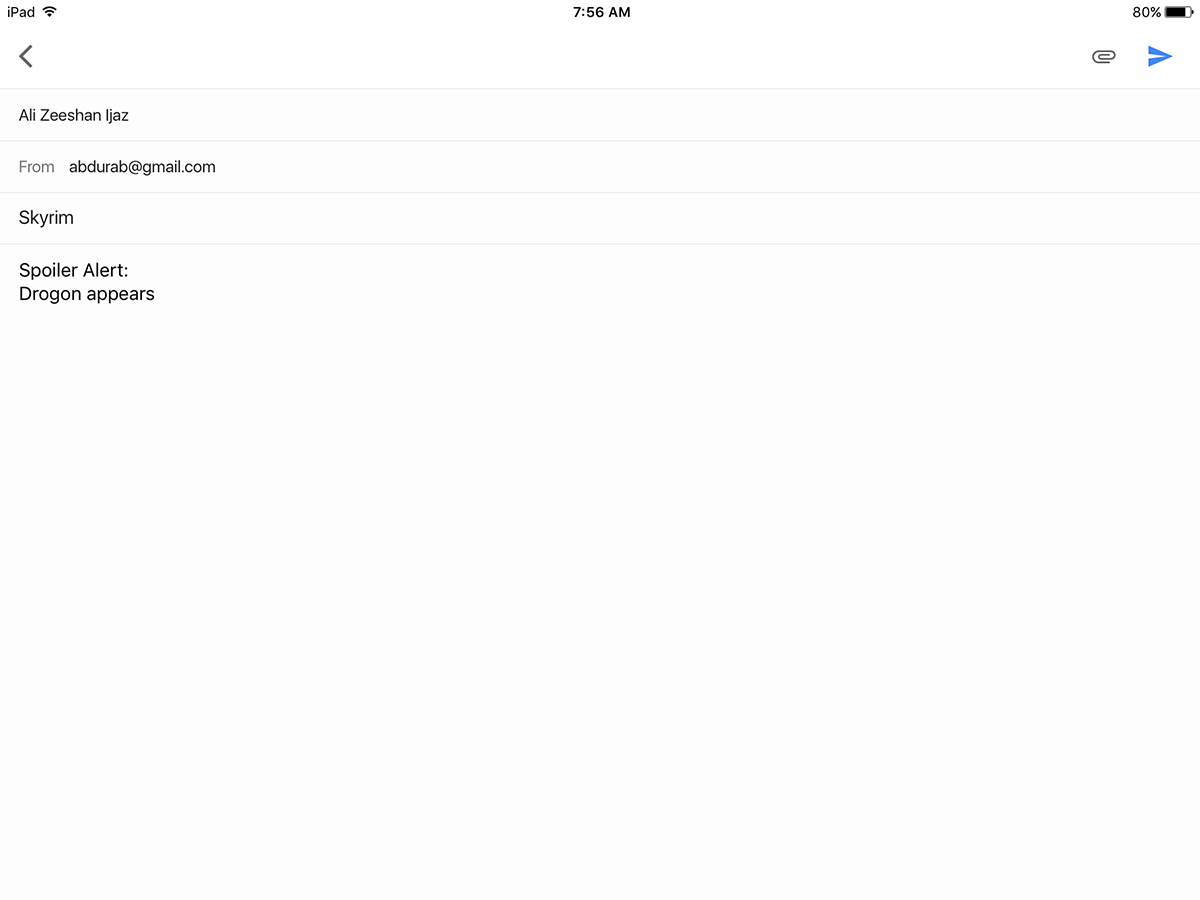The image depicts an iPad screen against a white background. At the top of the iPad, the status bar reads "7:56 AM" with the battery level at 80%. On the left side, there is a left arrow icon, and on the right side, there is a right arrow icon accompanied by a small paperclip icon.

Beneath the status bar, the text displays "All Zizan Legaz," followed by an email "from abderab@gmail.com." Below the email, the subject line reads "Skyrim," with a note underneath: "Spoiler alert: dragon appears."

The overall impression is that someone has received an email notification on their iPad early in the morning, letting them know about an anticipated plot point in the game Skyrim, specifically the appearance of a dragon.